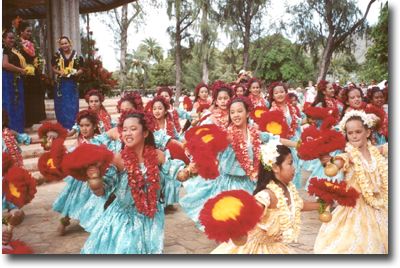This horizontally aligned image captures a lively Hawaiian luau, seemingly set in the 1960s or 70s, characterized by the participants' attire and style. The scene is outdoors under a mostly clear, slightly overcast sky, with verdant trees and palm trees providing a tropical backdrop. The ground appears to be dirt, lending a rustic feel to the festivities. 

At the center and right of the image, a group of women, clad in blue dresses and adorned with red leis, vibrant head decorations, and holding red and yellow pom-poms that resemble flowers, perform a synchronized dance. Their poses are dynamic, with legs outstretched and bodies crouching, capturing the energy of the moment. Accompanying these women are children in the lower right, dressed in gold-colored dresses with white flowers in their hair and gold leis around their necks, also holding red and yellow flower-like pom-poms, and following along with the dance.

In the upper left, several adult women are visible, wearing long blue skirts, black or dark blue tops with Hawaiian prints, and yellow leis. They stand on what appears to be a staircase or steps, contributing to the layered composition of the scene. Among them are three men dressed in blue wraps around their waists and black shirts with floral prints, playing ukuleles and singing, adding a musical element to the celebration.

Altogether, the vivid details of the attire, the lively movements of the dancers, and the natural setting create a vibrant portrayal of this traditional Hawaiian celebration.